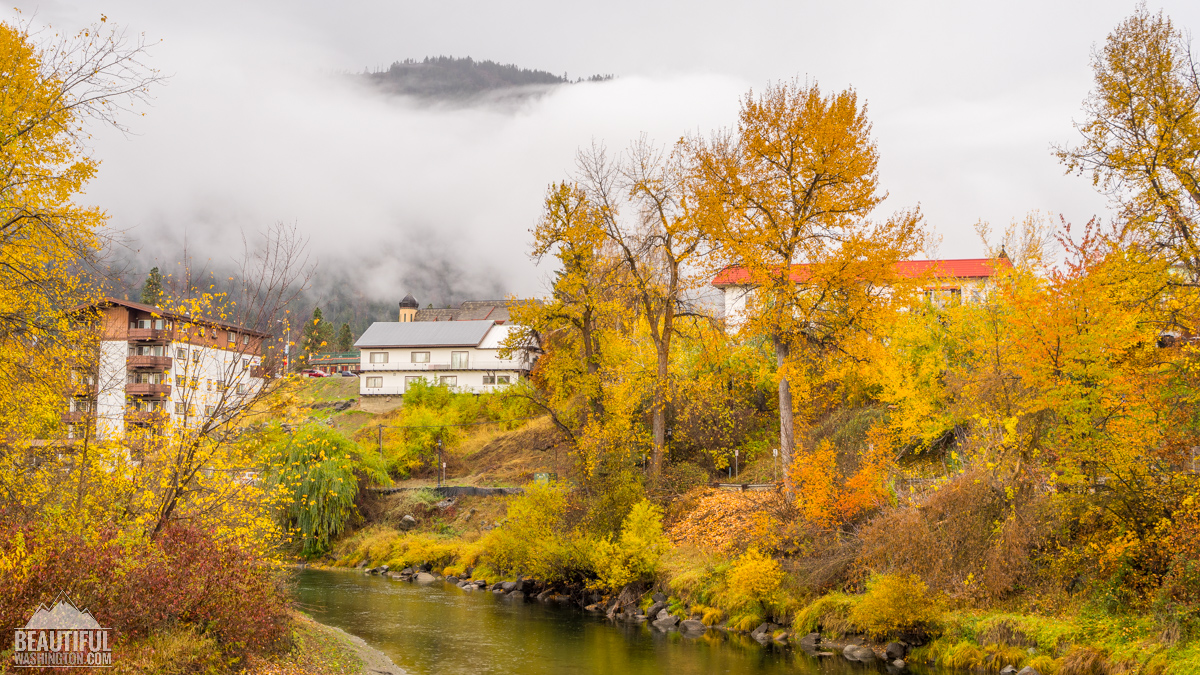The photograph depicts a small creek winding through a quaint, European-style town with residential properties perched above the riverbank. The scene is distinctly autumnal, with trees along the riverbanks displaying a vibrant mix of orange, yellow, and green foliage. Mist or fog casts an ethereal veil over the landscape, partially obscuring the distant mountain range, though one grassy peak manages to break through the mist. In the foreground, to the bottom left, there is a watermark for beautifulwashington.com. The properties along the river include buildings with various colored roofs—red, gray, and brown—with some featuring windows and balconies, hinting at an almost apartment-like or hotel appearance. The riverbanks are lush with trees, bushes, and a rocky shoreline, with a concrete walking path about 10 feet up the bank, weaving through the thick vegetation.